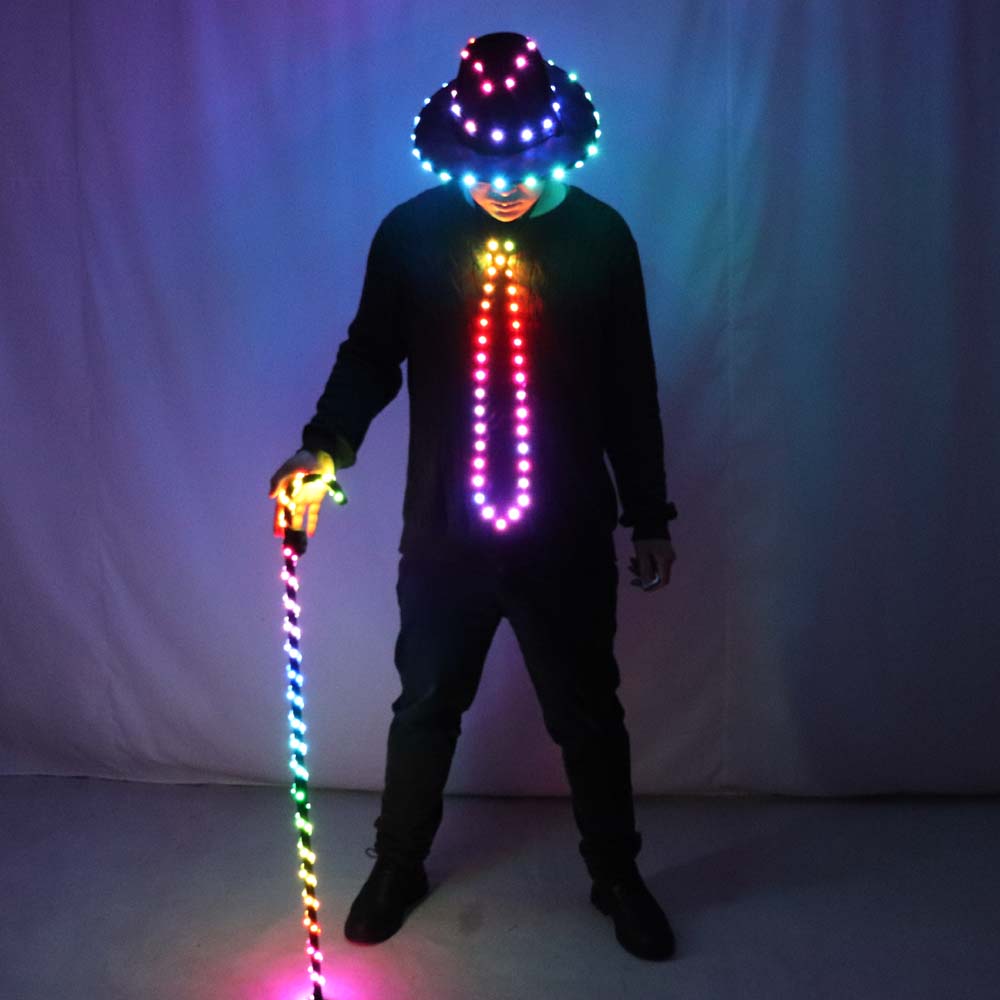In this highly detailed image, a person is dressed in an all-black ensemble, featuring a long-sleeve shirt, long pants, black shoes, and black gloves. They are also wearing a distinctive black hat adorned with multiple rows of glowing lights: blue lights circle the brim, red lights line the top, and purple lights can be seen as well. The person's head is bowed slightly, showcasing the illuminated hat.

Adding to the striking appearance, the person wears a light-up tie, with yellow lights at the top transitioning through red, pink, and purple hues down the length. The cane in their right hand, also wrapped in lights, complements this colorful theme. The lights spiral from purple at the top through blue, yellow, and red, ending in magenta at the bottom.

The background comprises a purplish drape or curtain with noticeable wrinkles, illuminated by the vibrant lights from the outfit, which adds depth and visual interest to the setting. The image captures a unique blend of colors and an eccentric, luminous style set against a concrete floor.